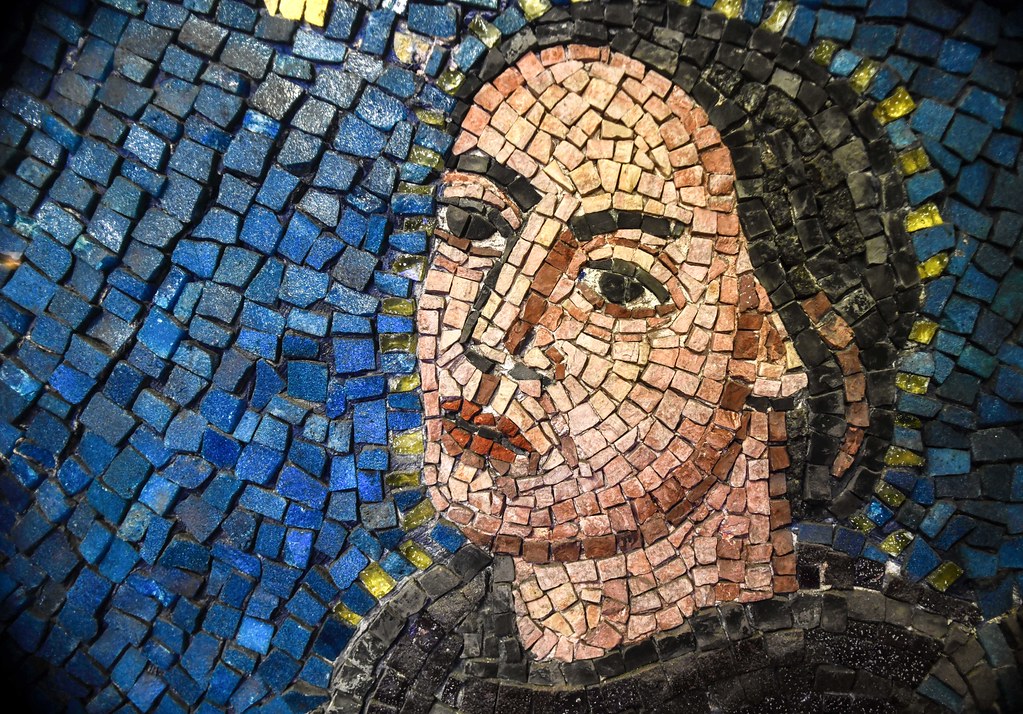The image is a detailed collage mosaic composed of small, mostly square but some irregular, tiles made of blue, black, yellow, tan, and rust-colored stones. Predominantly, the blue stones form the background and the edges of the artwork. The centerpiece of the mosaic is a depiction of a woman whose face and shoulders dominate the right side of the image. Her hair, appearing dark and possibly styled into a black hat, frames a face characterized by dark eyebrows, striking dark eyes, and rust-colored lips. Her skin is depicted in tan stones, and she wears a black robe. The tiles creating her image blend in square and occasionally broken shapes, while the surrounding blue and yellow stones provide a halo effect around her head, hinting at a possible religious context. The left side of the mosaic consists mainly of blue tiles, enhancing the contrast and emphasizing the woman's serene and contemplative expression as she gazes slightly to the left towards the viewer.